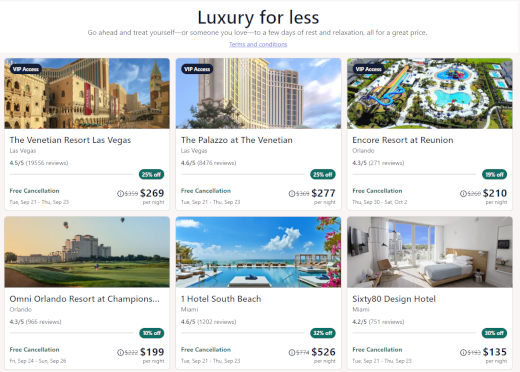Here's a detailed and cleaned-up caption for the image of the website describing various hotel-style destinations and resorts:

---

The image displays a website promoting various luxurious hotel and resort destinations against a clean, white background. At the top, bold black lettering prominently announces, "Luxury for Less." Below, a friendly message encourages visitors to "Go ahead and treat yourself or someone you love to a few days of rest and relaxation, all at a great price." In blue text, there's a clickable link labeled "terms and conditions" for further details.

The webpage features a series of hotels and resorts with accompanying images and brief descriptions. These include:

1. **The Venetian Resort Las Vegas**:
   - Located in Las Vegas
   - Rated 4.5 out of 5 stars
   - Reviewed by 19,556 guests
   - Offers free cancellation
   - Priced at $269 per night with a 25% discount

2. **The Palazzo at the Venetian Las Vegas**:
   - Rated 4.6 out of 5 stars
   - Priced at $277 per night with a 25% discount
   - Free cancellation included

3. **Encore Resort at Reunion Orlando**:
   - Rated 4.3 out of 5 stars
   - Priced at $210 per night with a 19% discount
   - Free cancellation included

4. **Omni Orlando Resort at Champions Orlando**:
   - Rated 4.3 out of 5 stars
   - Priced at $199 per night with a 10% discount

5. **One Hotel South Beach Miami**:
   - Rated 4.6 out of 5 stars
   - Priced at $526 per night with a 32% discount

6. **6080 Design Hotel Miami**:
   - Rated 4.2 out of 5 stars
   - Priced at $135 per night with a 30% discount

The website’s design highlights the irresistible offers, helping potential guests easily compare and choose their ideal luxury getaway.